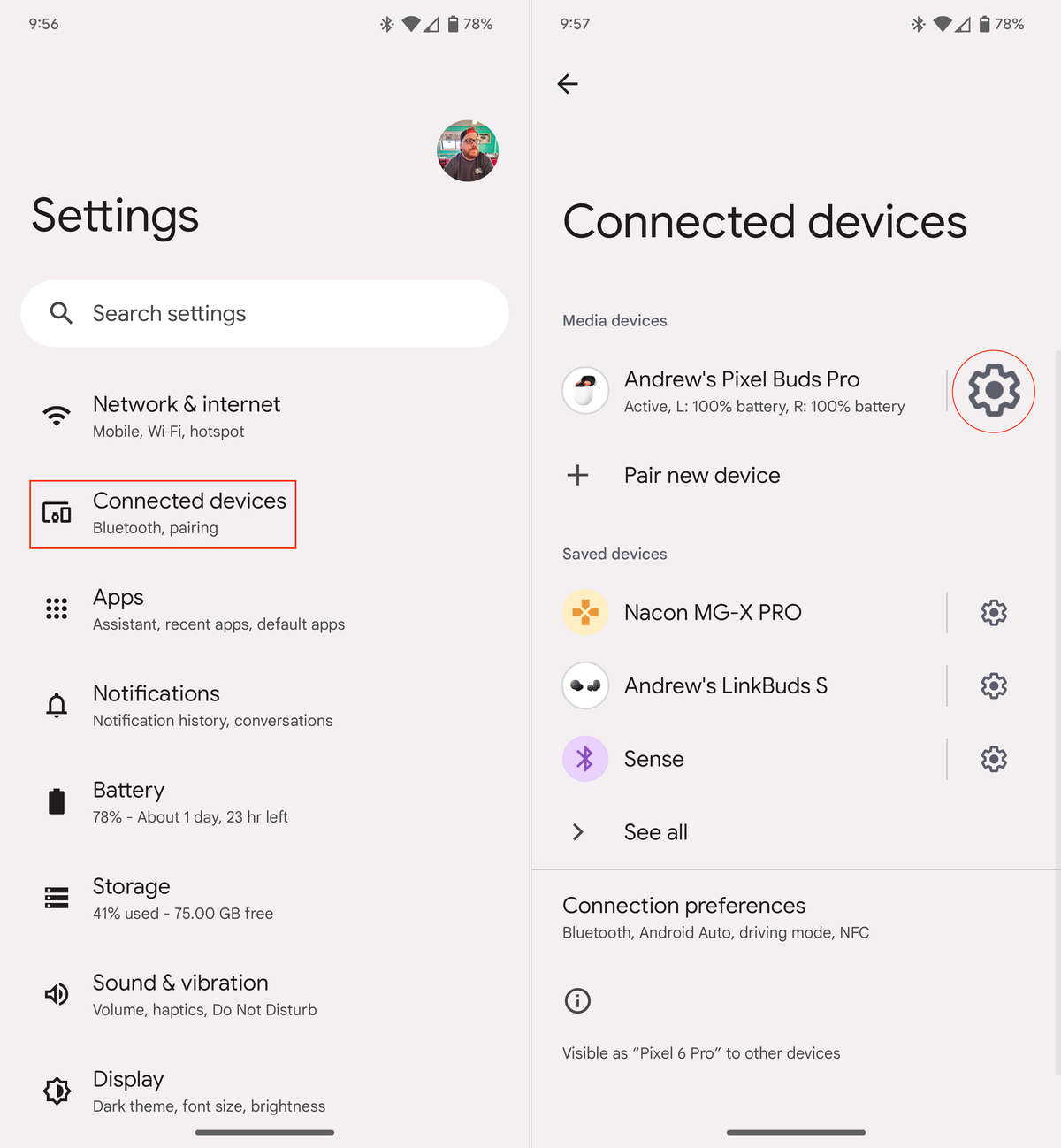Screenshot of a mobile device settings page with a gray/off-white background. The top of the screen displays the time as "9:56" on the left, along with icons for Bluetooth, Wi-Fi, data, and battery life at 78% on the right. Below this, the page title "Settings" is shown, accompanied by a search bar labeled "Search settings."

The menu items listed are:
- **Network & internet**: Mobile, Wi-Fi, Hotspot
- **Connected devices** (highlighted with a red box): Bluetooth, Pairing
- **Apps**: Assistant, Recent apps, Default apps
- **Notifications**: Notification history, Conversations
- **Battery**: 78%, About 1 day and 23 hours left
- **Storage**: 41% used, 75.00 GB free
- **Sound & vibration**: Volume, Haptics, Do not disturb
- **Display**: Dark theme, Font size, Brightness

On the right side of the screenshot, a submenu for "Connected devices" is opened. It shows:
- **Media devices**: Andrew's Pixel Buds Pro (active, left 100% battery, right 100% battery) with a red circle around a settings cogwheel.
- **Pair new devices**
- **Saved devices**:
  - Nacon MGX Pro
  - Andrew's Link Buds S
  - An option to "See all"

Lastly, under "Connection preferences," the options listed are:
- Bluetooth
- Android Auto
- Driving Mode
- NFC
- Visibility status as "Pixel 6 Pro" to other devices.